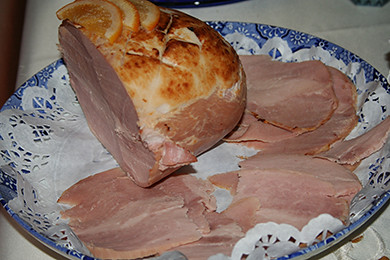A low-resolution, color photograph captures a tantalizing display of ham on a blue ceramic serving platter adorned with intricate white and dark blue flower patterns. The landscape-oriented image showcases the end piece of the ham, rounded side facing right and the cut facing left, near the top of the photo. The ham has been sliced thinly and meticulously arranged on a white paper doily that matches the size of the plate, featuring a delicate lacy border. The centerpiece of the display is a large segment of ham, garnished with vibrant orange slices, suggesting it has been glazed with an orange flavor. Surrounding the central piece are numerous uniformly thin slices of ham. The plate rests on a white tablecloth, with hints of additional plates barely visible at the top edges. The photo's realistic representation emphasizes the succulent and high-quality appearance of the ham, evoking a mouthwatering response.